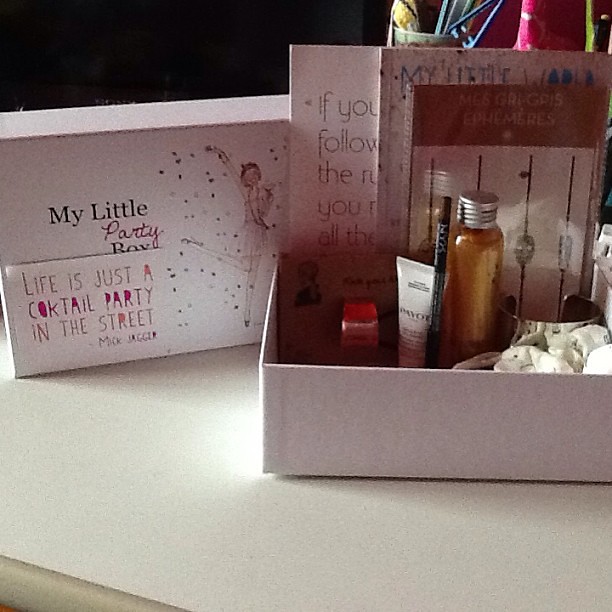The image displays two cardboard boxes on a white table against a solid black background. The box on the left is positioned behind the one on the right and is closed. It is white and features a whimsical cartoon illustration of a female dancer with long arms raised and one leg sticking out to the left, surrounded by confetti. Next to the dancer, the text reads "My Little Party Box," and underneath is a quote: "Life is just a cocktail party in the street." – Mick Jagger.

The box on the right is open, exposing various items inside. In the center sits an amber-colored bar with a silver cap. Adjacent to it, in the middle left section, there's a white squeeze bottle with black text, and a smaller bottle with a dark red cap is positioned lower. Three cards are propped up at the back of the box; the foremost card has a brown rectangular header with a pattern of white and brown vertical lines. The partially visible words on the card behind read, "if you," "follow," "the," and "you." The setup on the white surface is brightly illuminated, casting shadows from the boxes, which accentuates the depth and creates a clear visual contrast.